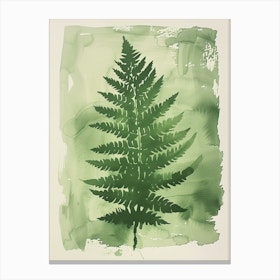The image depicts a detailed watercolor painting of a single, large fern leaf on a rectangular canvas with a white and tan border. The prominent fern leaf, rendered in dark green, stretches from the bottom of the image, where the stem starts, to the top, displaying an authentic replication of a real fern leaf found in nature. The leaf's shape features numerous smaller leaves that become longer towards the middle and taper off to a point at the top. Surrounding the fern is a rich green ombre background, with hues ranging from light pale green to darker shades of green and olive. This background is applied in a somewhat irregular, textured manner, adding to the rustic charm of the piece. The fern leaf is centrally positioned, with the watercolor creating a visually appealing frame that accentuates the natural beauty of the leaf.